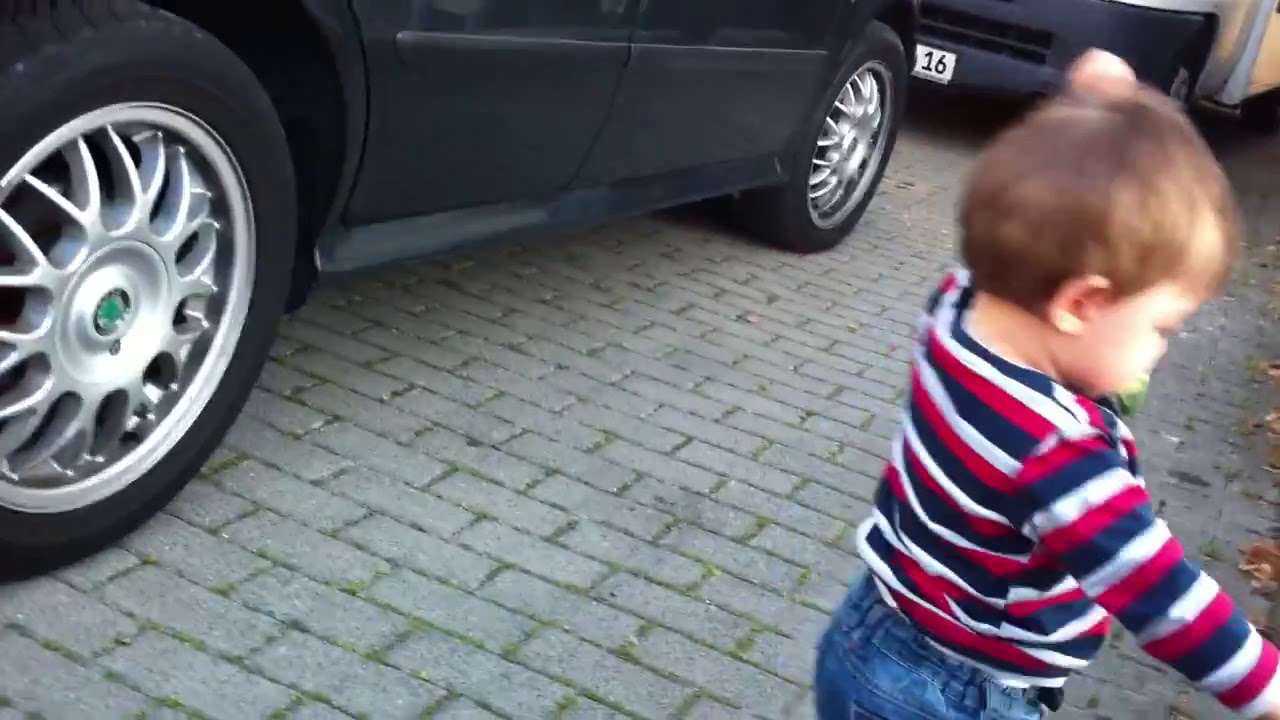This image captures a small, blurry toddler appearing to walk or stand on a driveway made of brick pavers with grass interspersed between them. The child's attire includes a long-sleeve shirt with blue, red, and white stripes, and blue jeans. His light brown hair and a glimpse of a green pacifier in his mouth are visible, and the image is cut off at his waist, leaving much of his lower body and one hand out of the frame. To the left, we see the lower portion of a black car, including its silver rims. Another car, also black, is partially visible in front of it. The top of the image cuts off parts of the scene, and scattered leaves are seen on the pavers to the right. In the top right corner is a white-yellowish blur. The main focus, however, remains on the toddler, who stands to the right side of the photo.